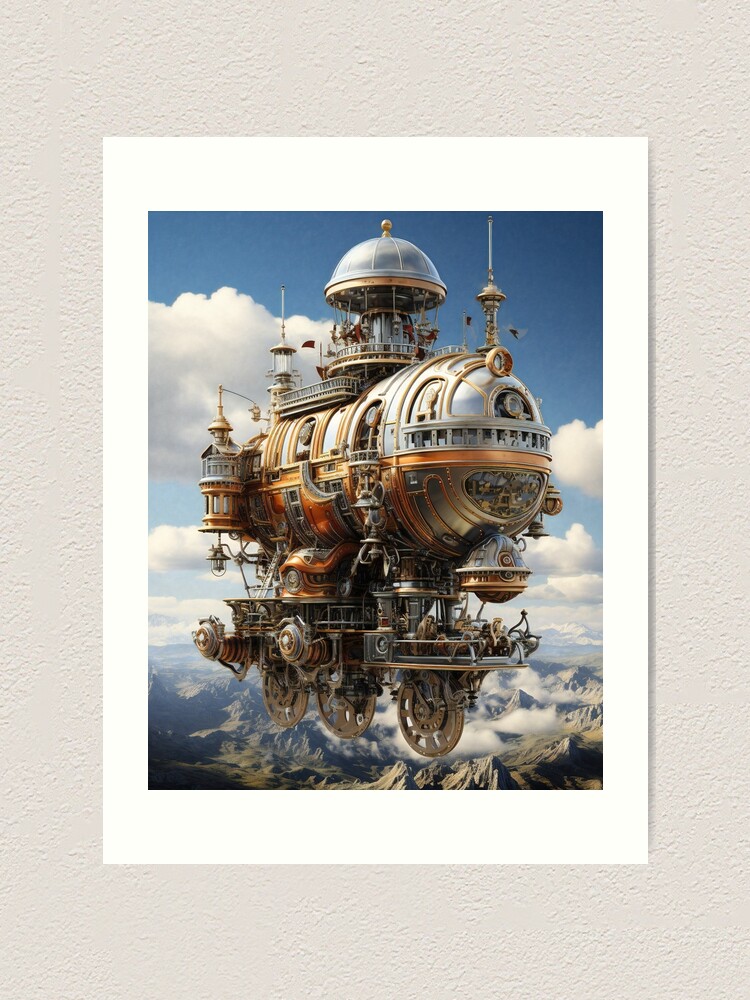This is an image of a computer-generated, futuristic flying machine displayed against a tan to white wall. The image has a white border and depicts a silver and copper-colored flying vehicle, shaped like an oval train cart with a gleaming metallic finish. This machine features a deck with people sitting on an outdoor balcony and boasts three silver wheels arranged from the back left to the front right, reminiscent of train wheels. The machine is designed with various gears and turrets, and it includes a carousel at the top with visible horses. It also includes skinny turrets, pointy antennas, a ladder, and a top tower with a rounded roof crowned by a gold piece. The detailed background reveals a blue sky filled with large, white clouds, with a mountain range showing dark brown and gray peaks shrouded in fog and clouds below the floating machine.